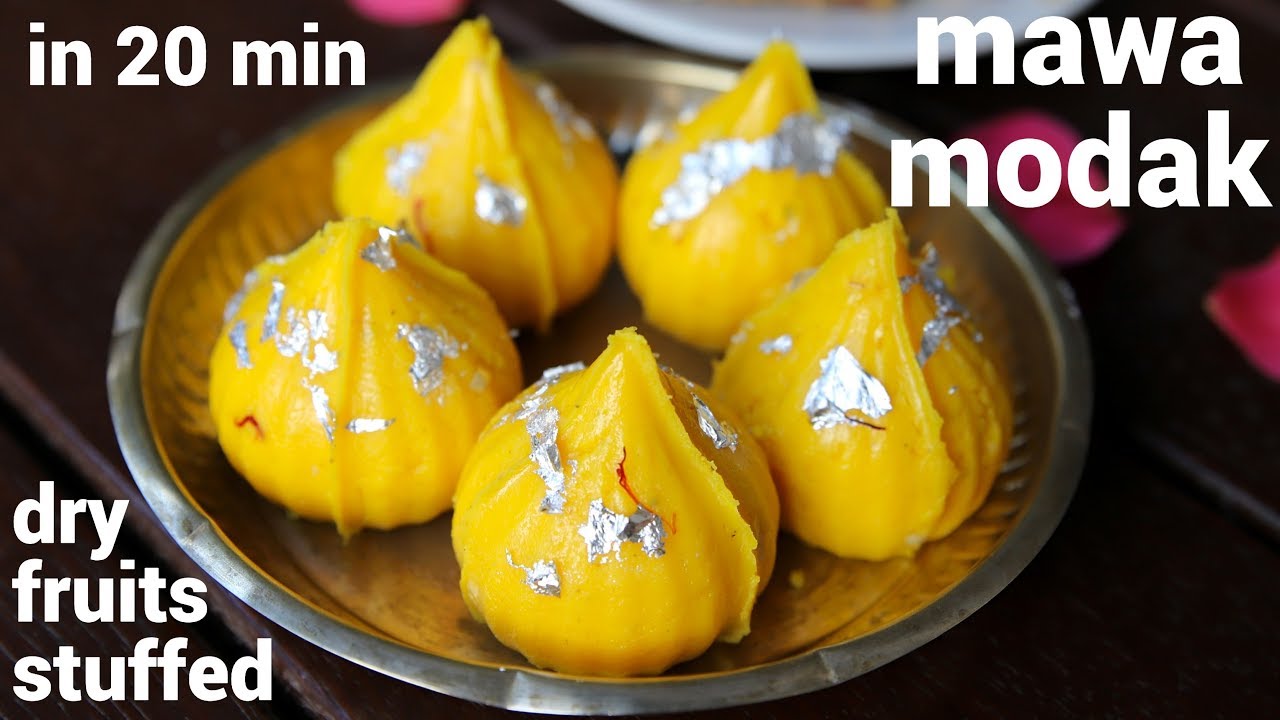The image is a photograph showcasing an advertisement for a recipe titled "Mawa Modak." The background features a dark brown or black surface, likely a dark wooden table. At the top center, a white round plate is partially visible, and on the upper left corner, the text "in 20 min" indicates the preparation time. On the right upper side, the white lettering spells out "mawa modak." 

In the foreground, a silver serving bowl presents four golden-yellow dry fruit-stuffed Mawa Modaks, each adorned with silver leaf and slight red accents. The Modaks have a distinctive bud-like shape, giving them an elegant appearance. To the right of the bowl, pink rose petals are scattered on the table, adding a touch of color and sophistication to the composition. At the very bottom left corner, the text "dry fruit stuffed" provides a brief description of the dish.